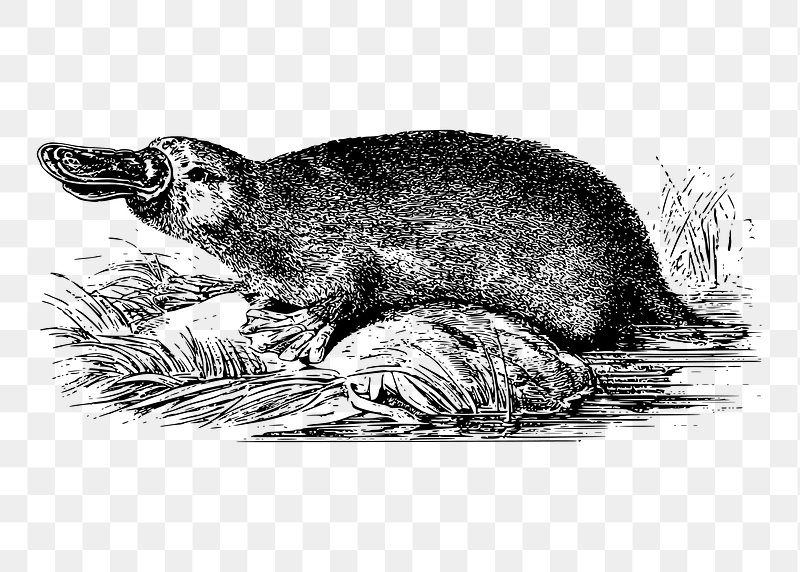This black and white line art illustration features a duck-billed platypus prominently positioned in the center against a transparent background, indicated by a gray and white checkerboard pattern. The landscape-oriented sketch shows the platypus with its distinctive elongated bill facing the left side of the image and its tail submerged in water on the right. The creature is depicted with webbed feet and short arms, partially emerged onto a grassy prominence surrounded by reeds or plants. This detailed depiction captures the platypus waiting or posing in a water setting, blending elements of both land and aquatic habitat.